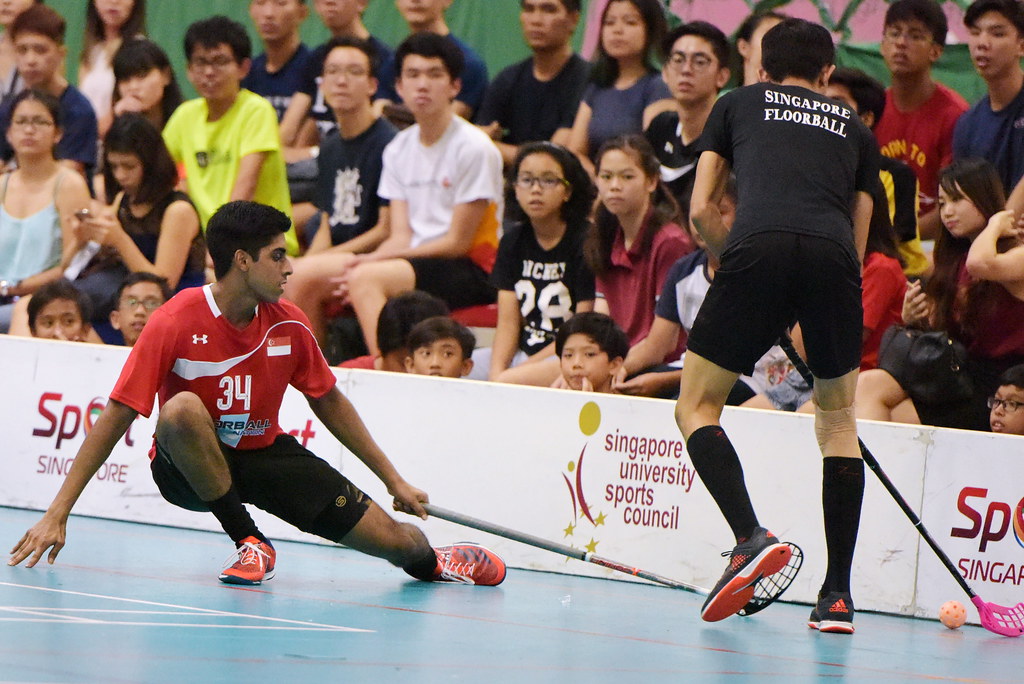The image depicts an intense floorball game in Singapore, as indicated by several banners displaying "Singapore University Sports Council" and "Sports Singapore." The court is smooth and bluish with white lines. Two main players are focused in the shot: one is dressed in a black shirt emblazoned with "Singapore Floorball" on the back, black shorts, and high black socks with sneakers. The other player sports a red uniform with the number 34, black shorts, high black ankle socks, and orange shoes. Both athletes wield floorball sticks, which look like streamlined golf club handles ending in plastic netted paddles. They're engaged in a tussle for a light pink wiffle ball. Spectators of various ages, including men, women, and children, watch the match from behind a perimeter marked by advertising banners.